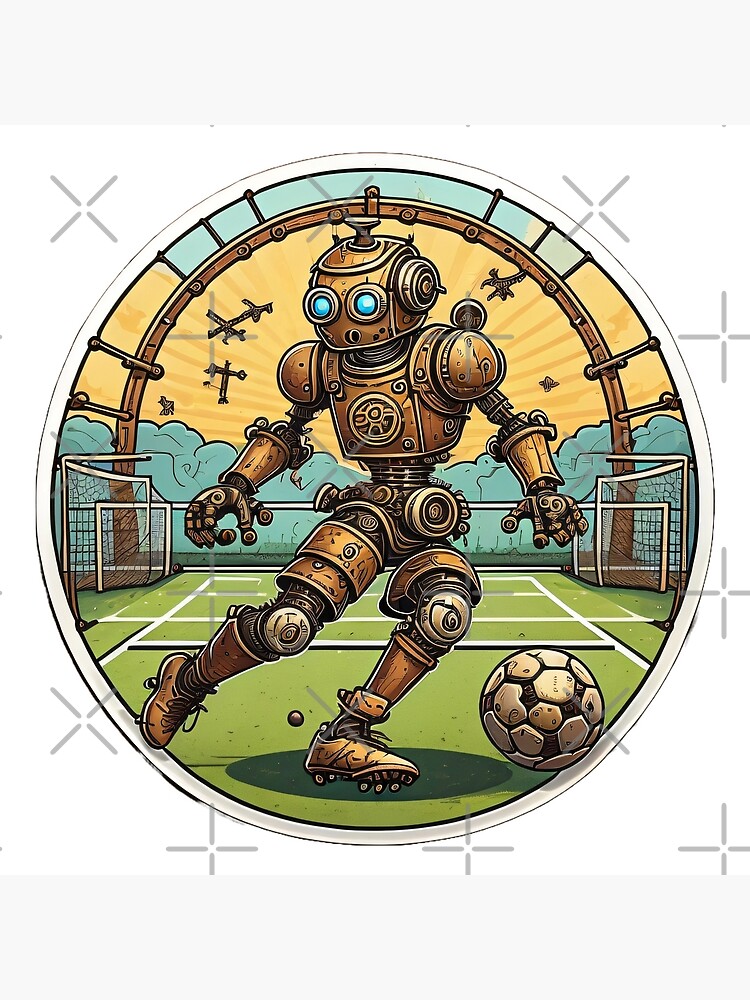The image features a detailed circular cartoon drawing centered on a dynamic scene of a robot playing soccer. The robot, primarily adorned in a striking gold and bronze ensemble, boasts bendable joints, gold-plated armor, wrist plates, cleats, and a headpiece with two large luminous blue eyes. The backdrop includes an expansive green soccer field marked with white lines and flanked by two white nets suggesting goalposts. Above, a golden sky populated with flying mechanical objects frames the scene. Encompassing this centerpiece are gray horizontal bars at the top and bottom of the circle, set against a white background interspersed with X's and plus signs. The robot, seemingly caught mid-action with hips swiveled to the right, appears poised to kick a golden and black soccer ball. All metal in texture, the scene exudes a futuristic yet playful essence, with blue clouds and stars accentuating the vibrant and spirited atmosphere.